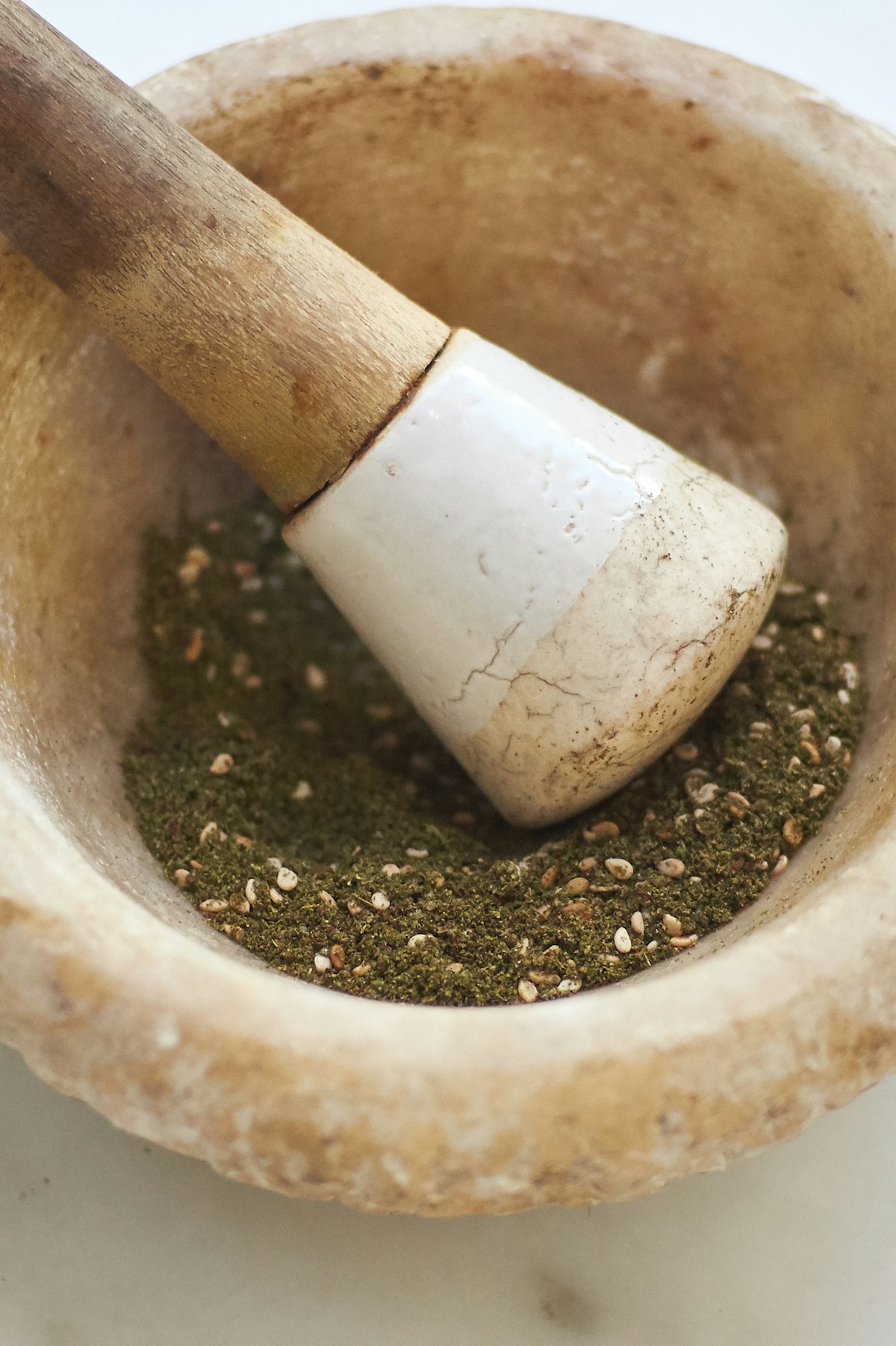The image showcases a well-worn, zoomed-in view of a wooden mortar and pestle, indicative of extensive usage over time. The mortar exhibits a light brown, almost bone color with slight discolorations, evidenced by dark brown and white spots that add to its aged appearance. The pestle, featuring a wooden handle darkened by years of absorbed oils, transitions into a white, ceramic-like tip marked with minor cracks and imperfections attesting to its frequent use. Nestled inside the mortar are finely ground herbs and seeds, highlighting the pestle's functionality as it rests against the side, blending seamlessly with the seasoned feel of both tools.